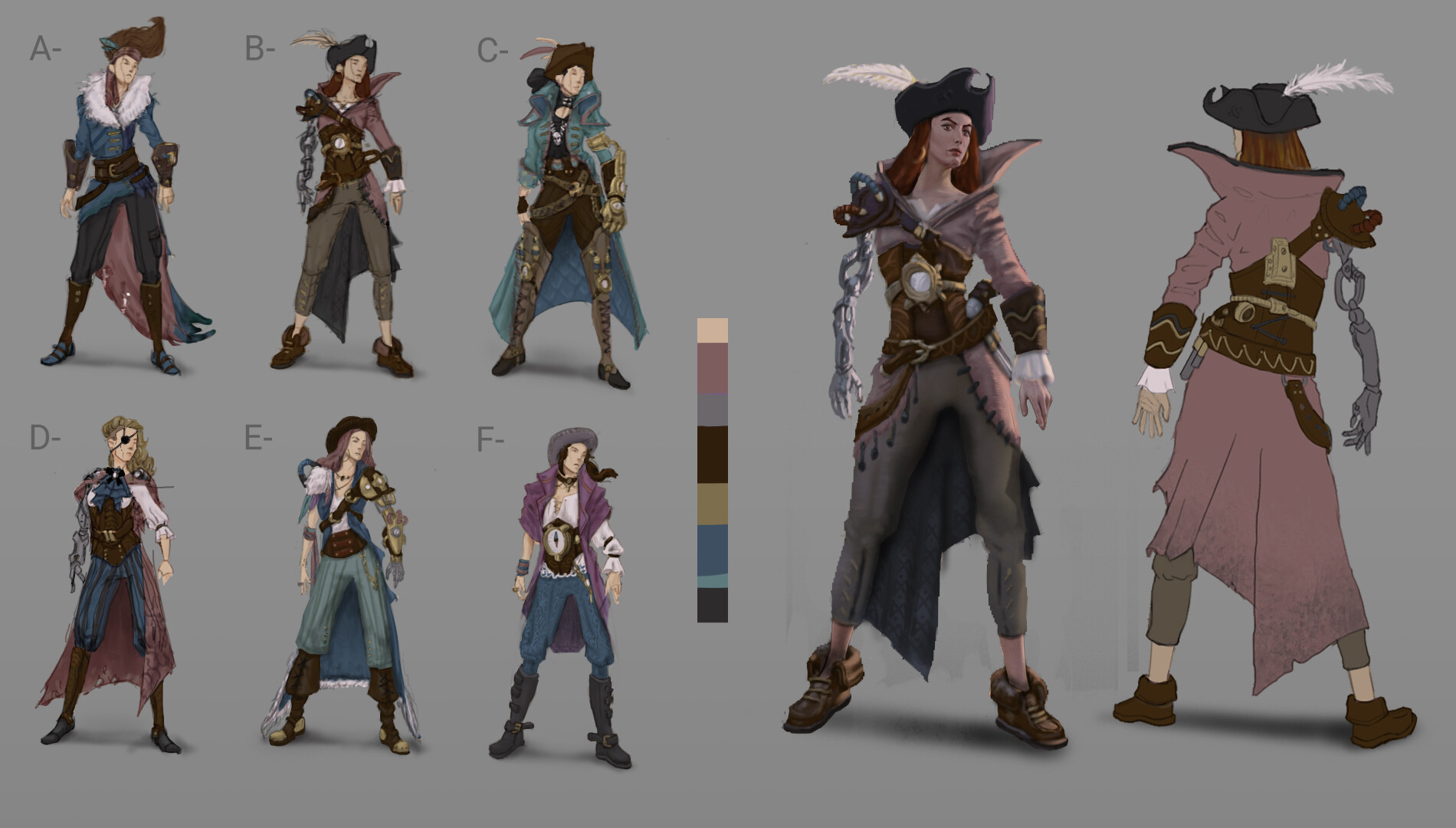This image showcases a series of eight CGI-rendered or cartoon-like concept art drawings featuring one or more women dressed predominantly in pirate-themed attire. These illustrations appear to be part of a character customization process, possibly for a video game, cartoon, or movie. Each character is adorned in various outfits, fitting within a specific color palette that includes shades of blue, brown, tan, dark teal, cream, mauve, gray, black, and gold. A striking feature across most of the illustrations is the presence of a metallic, robotic arm, indicating a blend of historical pirate aesthetics with advanced technology. 

The layout consists of six smaller figures on the left, labeled A through F, and two larger, more detailed images on the right, displaying the character from front and back. The character is seen wearing a pirate hat with a feather and some form of armor on her chest. Between the two sections of images is a small color block, showing the palette used for these designs. This collection of images likely represents different iterations or outfit options for a single female character, showcasing the creative process of determining her final look.